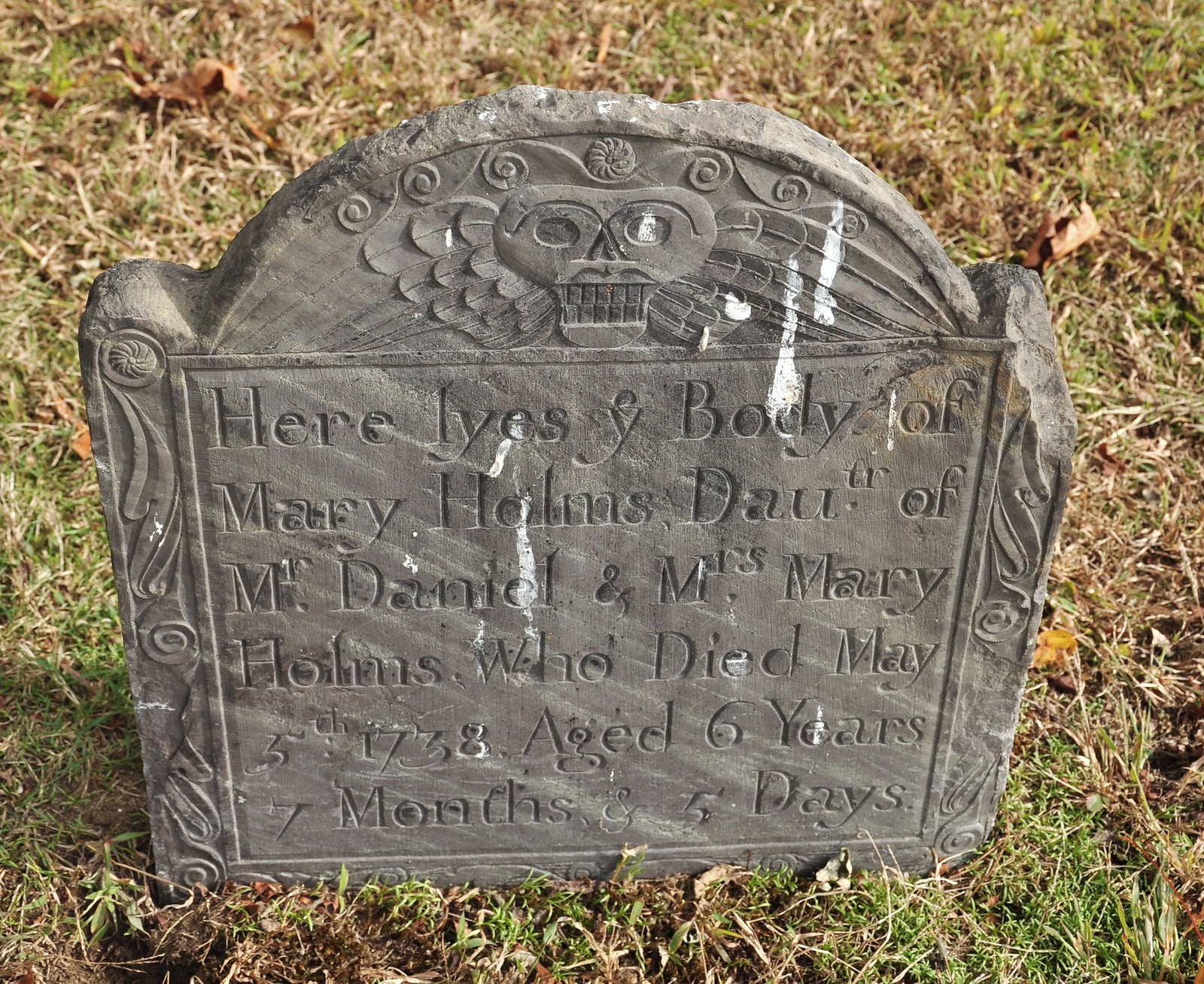The image depicts an outdoor scene featuring a historic tombstone set amidst dry grass with scattered patches of green and occasional dried leaves. The gray headstone, partly weathered and eroded, prominently displays bird droppings and boasts intricate detailing. Its upper section is adorned with a carved skull and scrolls, along with a depiction of two birds facing each other, showcasing their feathers. Decorative elements embellish the sides of the headstone, despite a noticeable break and jagged edge on the upper right corner. The central inscription, though aged, remains legible, reading: "Here lies the body of Mary Holmes, daughter of Mr. Daniel and Mrs. Mary Holmes, who died May 5, 1738, aged six years, seven months, and five days."